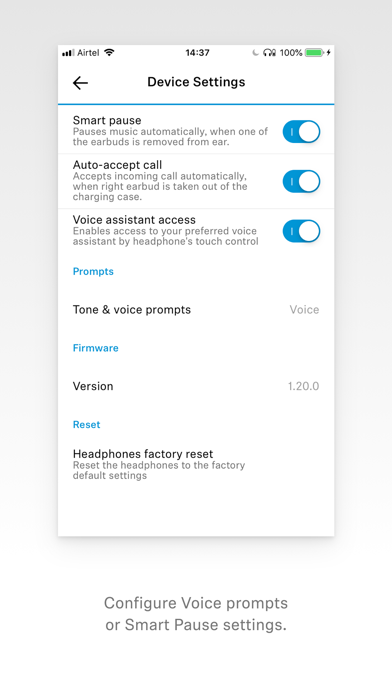The image displays a smartphone screen with a gradient gray-to-white background. At the top of the screen, "Airtel" is displayed between the internet strength bars on the left and the Wi-Fi strength bars on the right, with the time "14:37" centered and the battery power indicator on the far right.

Below this header, the text "Device Settings" is written in black with a blue underline. The settings are organized into three sections, each marked by a blue toggle button indicating they are enabled:

1. **Smart Pause**: Automatically pauses music when one of the earbuds is removed from the ear.
2. **Auto Accept Call**: Accepts incoming calls automatically when the right earbud is taken out of the charging case.
3. **Voice Assistant Access**: Enables access to the preferred voice assistant through the headphones.

Further details include the following elements mentioned underneath "Touch Control":

- "Prompts" in blue, followed by "Tone and Voice Prompts" in black.
- "Voice" in gray below the prompts section.
- "Firmware" in blue, followed by "Version 1.20.0" in black.
- "Reset" in blue, followed by "Headphones" in black text indicating factory reset options, explaining that it will reset the headphones to the factory default settings.

At the very bottom of the screen, in gray text, it reads: "Configure voice prompts or smart pause settings."